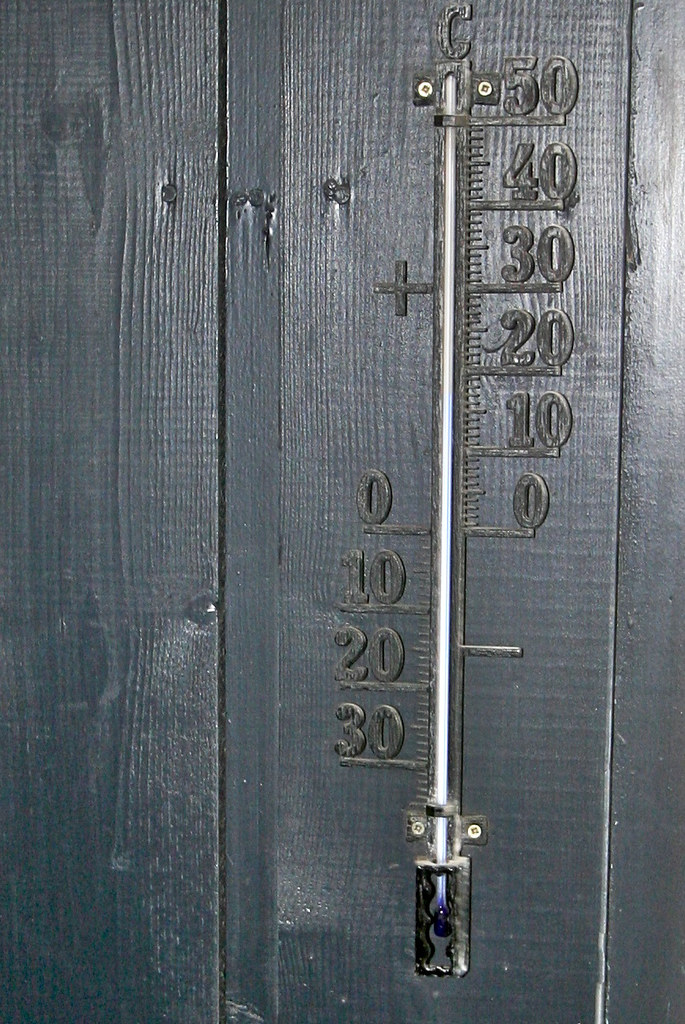This vertically-oriented color photograph captures a meticulously mounted metal thermometer affixed to a textured, dark blue-gray painted wooden wall. The thermometer is securely fastened with screw plates located at both its top and bottom. A prominent feature is a long metal piece at its center, housing a thin white glass tube that likely contains the measurement gauge.

At the base of the glass tube rests a round blue bulb. The thermometer displays temperature in both Celsius and Fahrenheit, with numerals etched on either side. The left side starts from 30°C, descending through 20°C, 10°C, and down to 0°C, all accompanied by precise line markings. Correspondingly, the right side mirrors the same 0°C mark in the center and ascends in Fahrenheit from 0°F to 50°F.

Highlighting the scale is a metallic letter 'C' positioned at the top of the thermometer, adding a distinct touch. The wooden wall or fence it is mounted on showcases visible wood grain and texture, enhancing the rustic feel of the image.